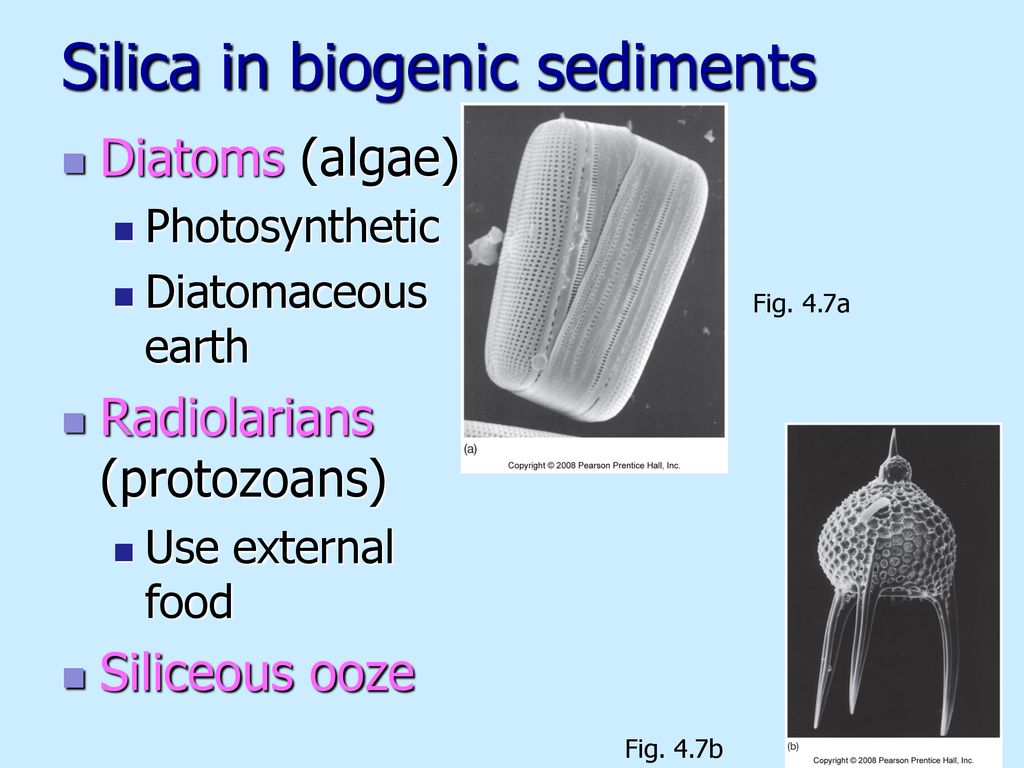**Detailed Caption**: 

**Silica and Biogenic Sediments**

- **Diatoms** (In pinkish-purple text)
  - (Algae)
  - Photosynthetic (In black text)
  - Diatomaceous Earth (In black text)

- **Radiolarians** (In pinkish-purple text)
  - (Protozoans)
  - Use external food (In black text)

- **Siliceous Ooze** (In pinkish-purple text)

**Figures:**
  - **Figure 4.7a**: Depicts a protozoan that has a somewhat rectangular shape. At the bottom of the figure, it states "Copyright 2008 Pearson Prentice Hall Inc."
  - **Figure 4.7b**: Shows an organism resembling a spore with three leg-like extensions or something akin to a Christmas ornament. This figure also includes the note "Copyright 2008 Pearson Prentice Hall Inc." in the bottom right-hand corner.